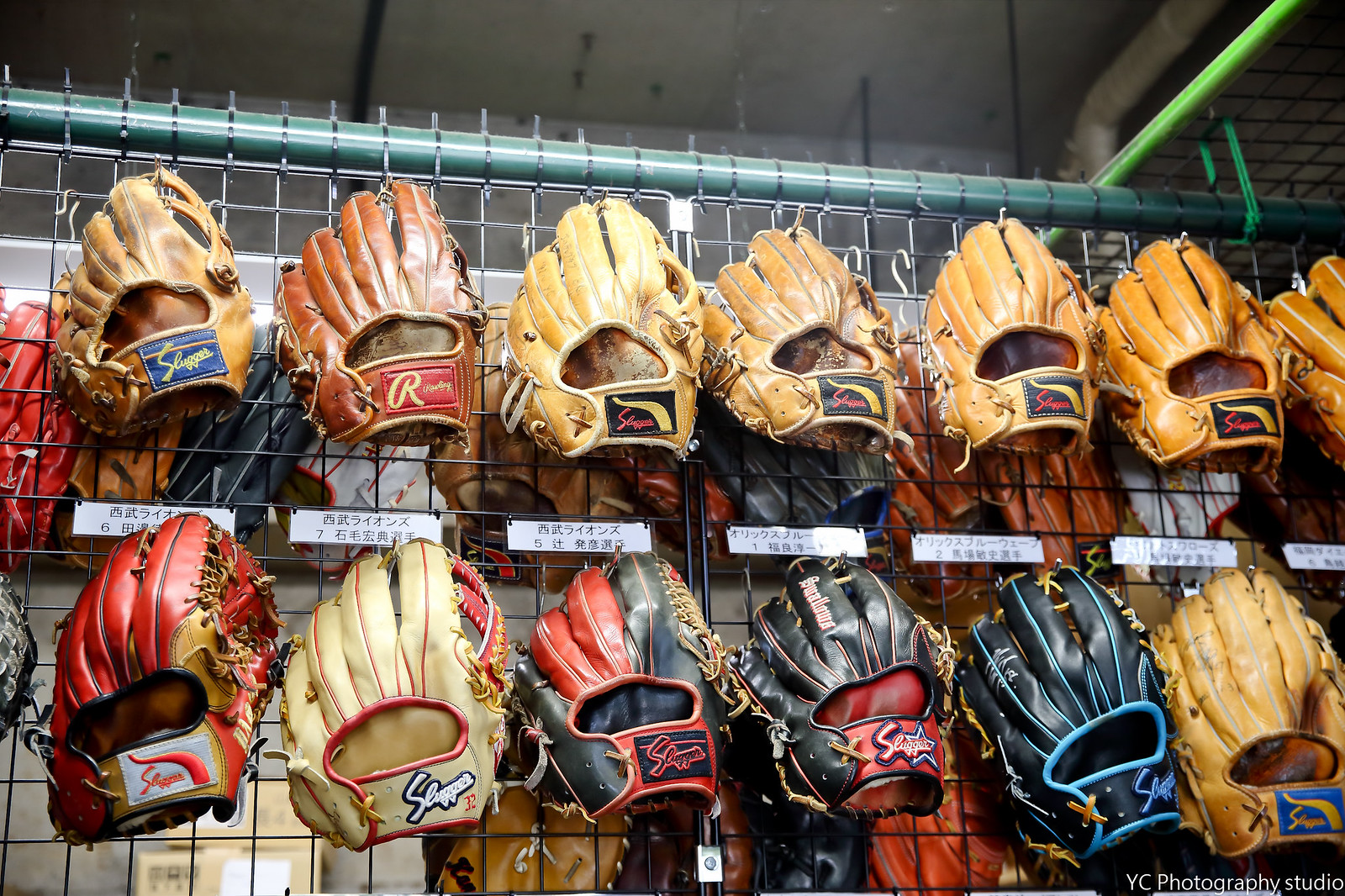This color photograph captures a detailed indoor display of 13 baseball mitts arranged meticulously on a wire mesh grid composed of 2-inch metal squares. The mitts, each distinct in color, range from shades of beige, brown, and tan to vibrant reds, blues, and blacks, with some featuring colorful linings and stitching. Each mitt hangs neatly in two rows – seven in the top row and six in the bottom – secured by S hooks to the wire grid, which itself is held up by black zip ties attached to a green metal bar linked to additional green supports. Below each mitt, small white placards featuring Japanese or Chinese text provide information, possibly indicating brand details or prices, contributing to a feeling of this being either a retail or collection display. The overall setting appears to be an indoor space with a gray ceiling visible at the top of the image. The bottom right corner of the photograph contains white text reading "YC Photography Studio," suggesting this is a professional photograph capturing the meticulous order and variety of the baseball mitts. Reddish hues visible through the grid hint at further gloves displayed on the other side, reinforcing the impression of a comprehensive and well-organized exhibit.